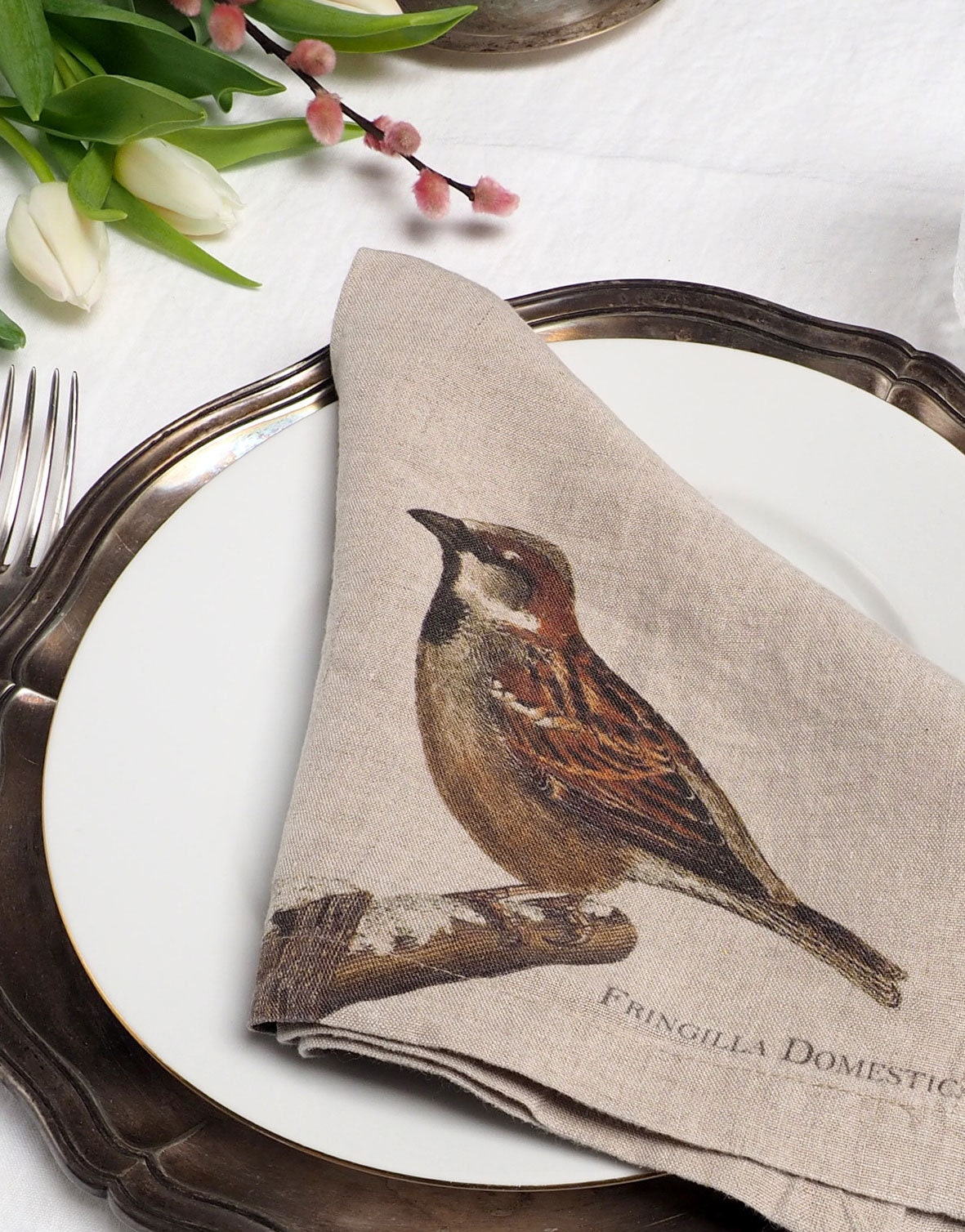In the photograph, a refined dining setting is captured, showcasing a brass, round silver tray that holds a round porcelain white plate, slightly off-center near the right and top of the image. A grayish-toned napkin, meticulously folded, partially covers the white plate, extending off the image at multiple points. Centered on the napkin is an exquisite illustration of a brown Fringilla domestica bird perched on a snow-dusted tree branch. The bird features a light brown belly, with darker brown underparts, a black and orange wing adorned with a touch of white, and tail feathers that transition from dark on top to gray underneath. Its distinguishing traits include an orangish hue above its eye, a short black beak, with some black and white detailing around its head. Below this delicate artwork, the napkin bears the text “Fringilla Domestica.” The scene is complemented by a floral arrangement at the top, comprising white unopened buds, green leaves, and slender branches with pink buds. A metal fork is positioned to the left of the napkin, partially out of frame, adding to the elegance of the setting, all displayed atop a white tablecloth.